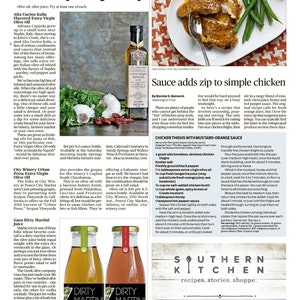The image depicts a magazine or newspaper page, featuring four distinct sections and one detailed recipe. At the top of the page is an image of a bottle of olive oil accompanied by onions and basil. Below this, there are two sealed glass bottles, partially labeled “dirty something” with the bottom part of the text obscured. 

In the top right corner, a photograph showcases a white oval plate on a tablecloth-covered table. The plate contains a serving of chicken alongside green beans, with a fork placed beside the food. Accompanying this picture, there is a story headlined, "Sauce Adds Zip to Simple Chicken," followed by the recipe presumably for the depicted chicken dish.

The bottom right corner of the page prominently displays the text "Southern Kitchen Recipe Stories Shop," affirming the layout's resemblance to a traditional magazine or newspaper rather than a webpage. However, the zoomed-in view makes some of the text blurry and unreadable.